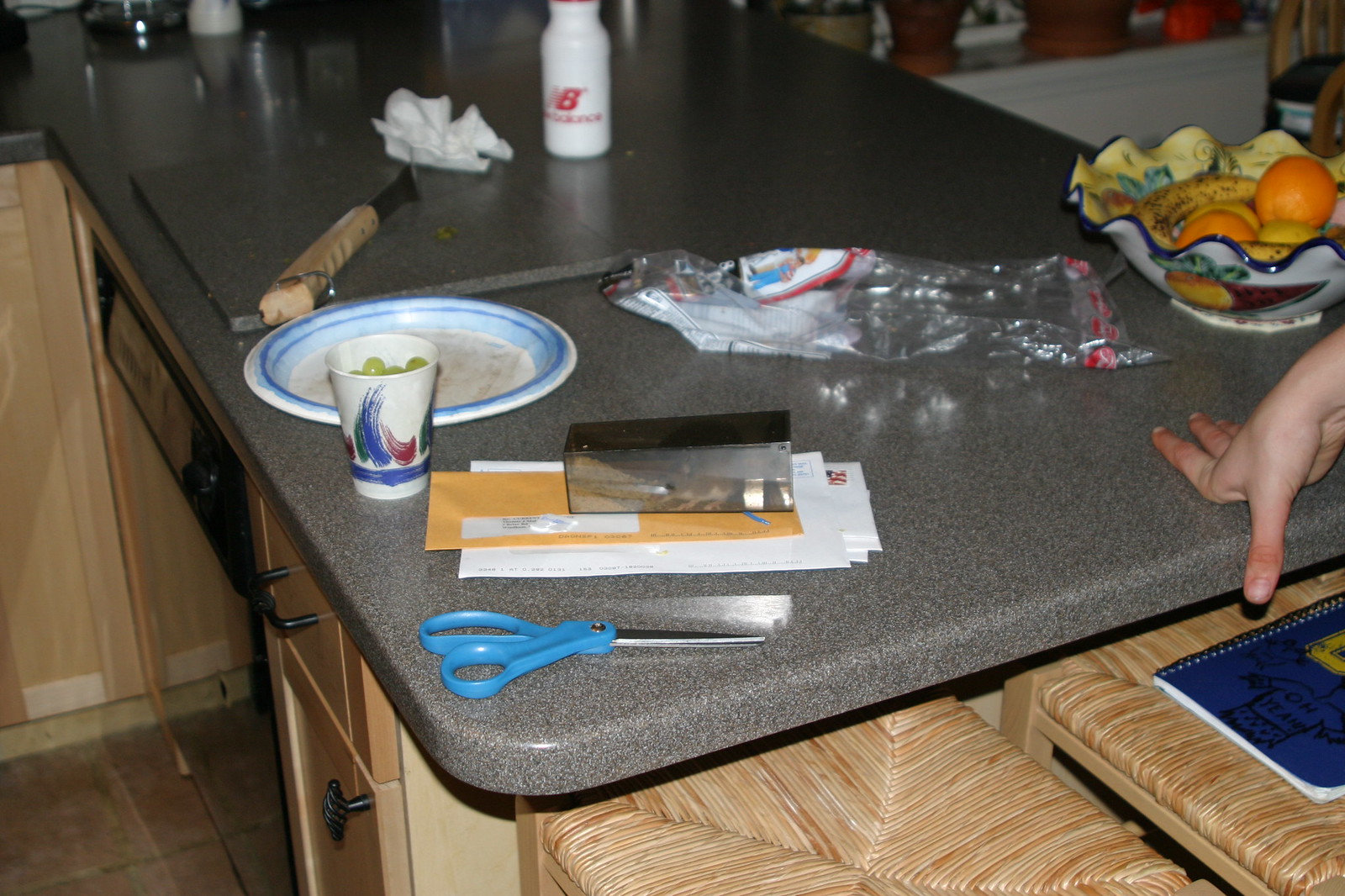In a cozy home kitchen, the gray countertop serves as a hub of activity, surrounded by barstool seating with wicker seats and blonde-colored wood, neatly pushed under the counter's lip. On the countertop, a variety of everyday items paint a vivid picture of daily life. A pair of scissors with blue handles lies next to a stack of mail, hinting at recent correspondence. A paper cup filled with grapes adds a touch of healthy snacking, contrasting with an otherwise empty bag nearby. A bowl of fruit takes center stage, though its bananas are noticeably overripe. A cutting board, still bearing traces of food debris, speaks of recent meal preparations, while a large fork for turning meat rests beside it. A wadded-up napkin or paper towel suggests a quick clean-up. A plastic reusable water bottle, the type that fits into a bike's water cage, stands ready for hydration. An anonymous hand reaches into the frame, touching the table, adding a human element. Underneath the countertop, on one of the stools, a wire-bound notebook lies, perhaps waiting for the next jotting of a grocery list or a recipe note.